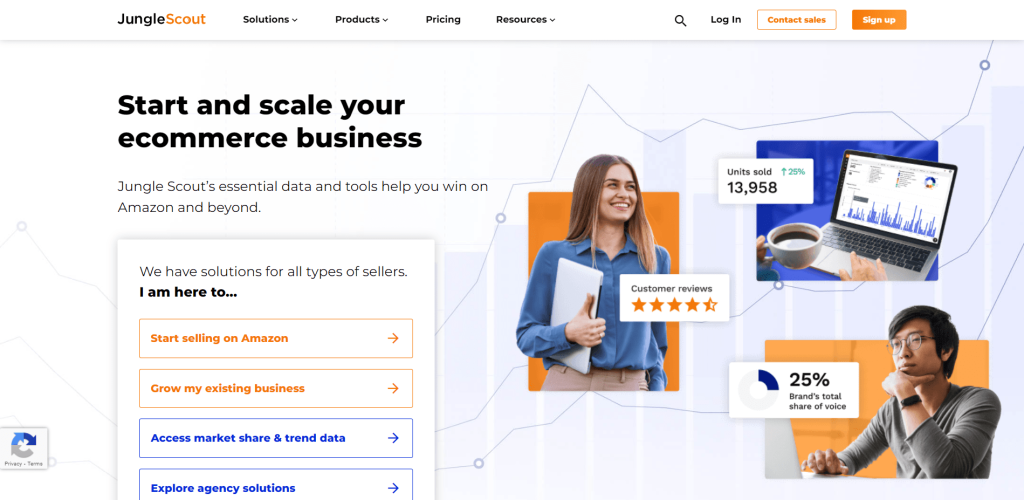This image showcases the Jungle Scout website's homepage. In the upper left corner, the "Jungle Scout" logo is prominently displayed, with "Jungle" in black font and "Scout" in an orange hue. Positioned along the top navigation bar, from left to right, are the menu items: "Solutions," "Products," "Pricing," and "Resources." Further to the right, there is a search magnifying glass icon, followed by options to "Log In," a "Contact Sales" button, and a "Sign Up" button.

Beneath this navigation bar lies the principal content of the homepage. On the left side, a headline reads, "Start and scale your e-commerce business," followed by smaller text stating, "Jungle Scout’s essential data and tools, helping you win on Amazon and beyond." Below this text, a white box offers four selectable options stacked vertically: "Start Selling on Amazon," "Grow My Existing Business," "Access Market Share and Trend Data," and "Explore Agency Solutions."

On the right side of the main section, there are three images arranged vertically. The first image features a woman holding a laptop, the second depicts a man seated and working on a laptop, and the third shows a laptop with a coffee cup entering the frame from the side.